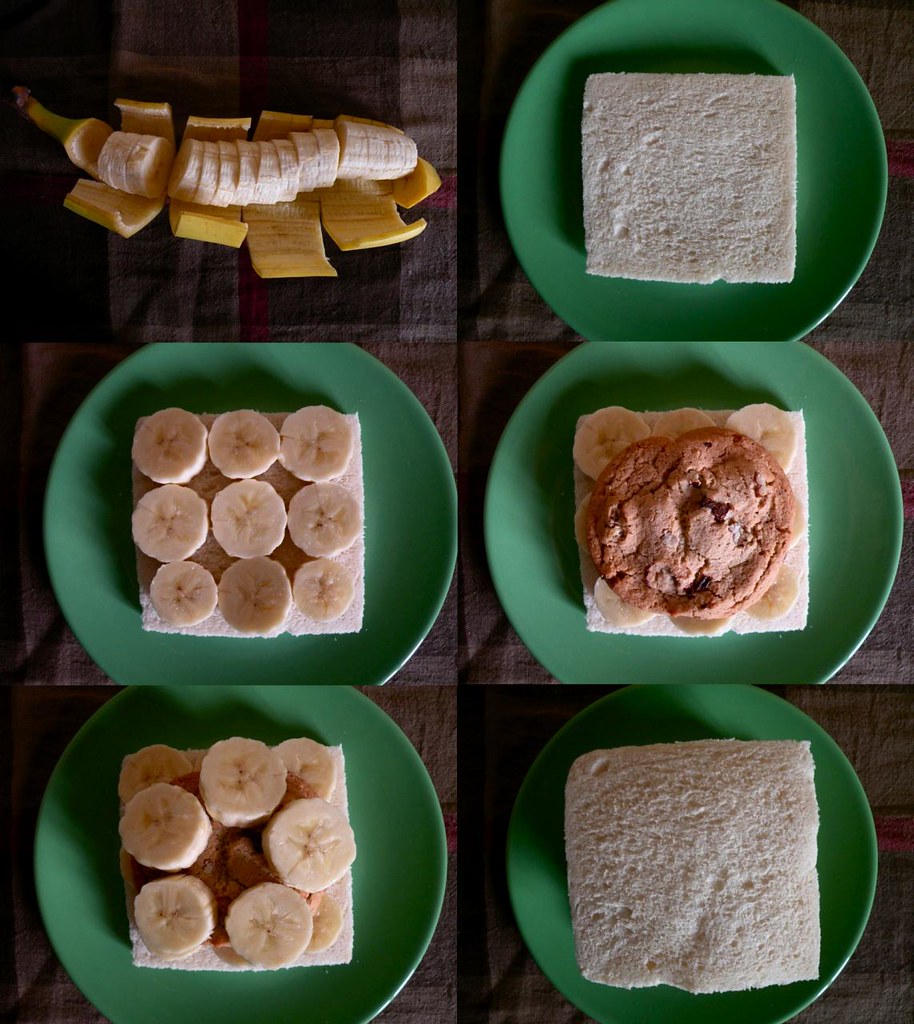The image features a collage of six realistic photos displayed in two columns and three rows, set against a wooden table background. 

In the top left, a banana is artistically sliced along with its peel, with the slices neatly arranged inside the partially opened peel. 

Directly below, two green plates showcase pieces of crustless bread: one with nine banana slices neatly arranged in rows, and the other with a layer of banana slices atop what appears to be peanut butter.

The right column consists of three green plates with square slices of crustless bread. The top and bottom plates display plain bread slices, while the middle plate has a cookie placed on top of the bread.

This detailed arrangement visually documents the process of creating a banana and peanut butter sandwich, with the final image in the sequence showing the completed sandwich with only the top slice of bread visible.